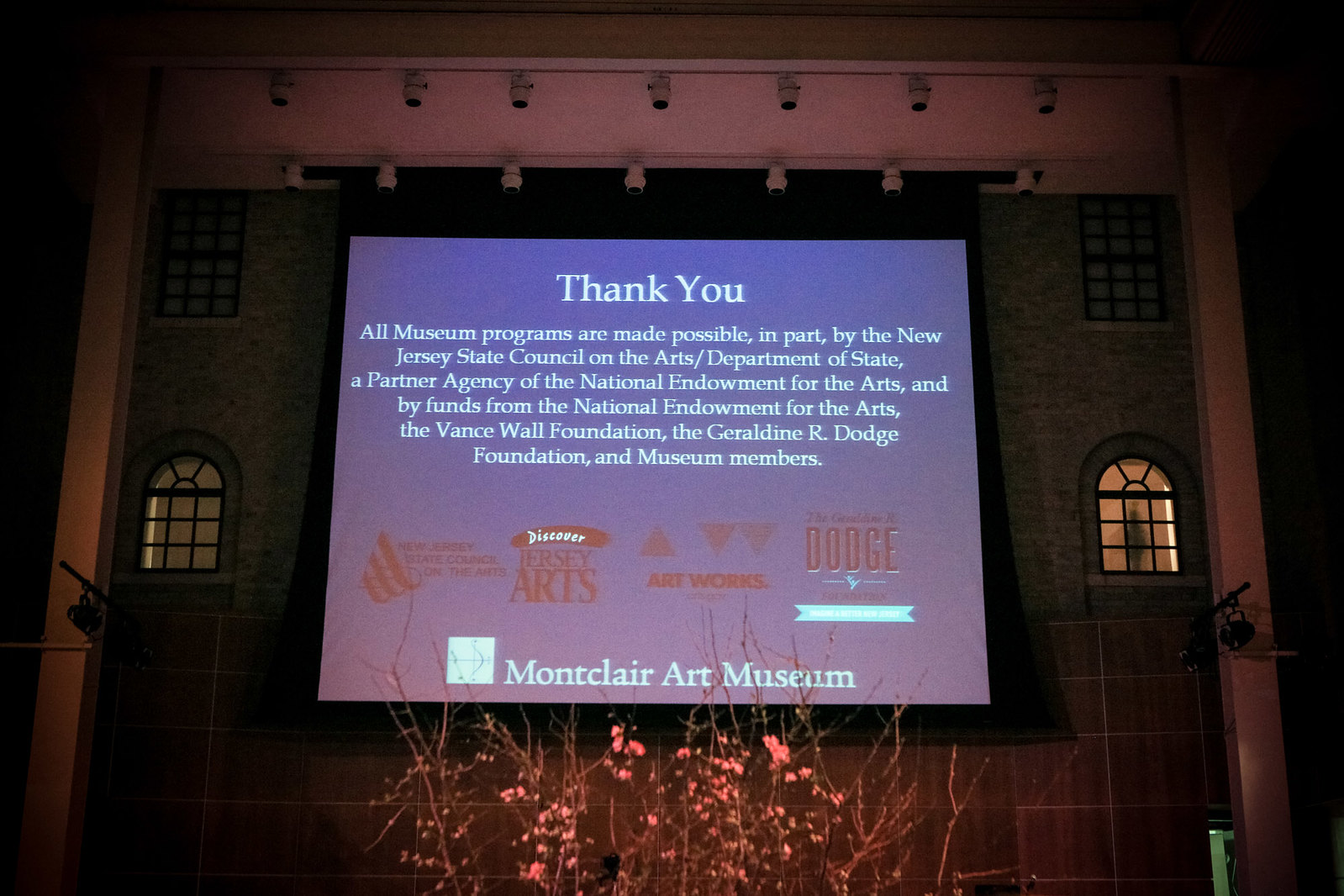The image shows a large rectangular projection screen set against a stage background designed to resemble the side of a building, with sage green walls and black-edged, curved rectangular windows, complemented by brown tiles at the base. The stage is darkly lit and features white cylindrical theater lights above the stage, which are turned off. On the screen, which has a black border, a slide with a blue background is projected. The slide's white text at the top reads "Thank You." Following this, in smaller white font, it states that all museum programs are made possible in part by the New Jersey State Council on the Arts/Department of State, a partner agency of the National Endowment for the Arts, and by funds from the National Endowment for the Arts, the Vance Wall Foundation, the Geraldine R. Dodge Foundation, and museum members. The slide also includes multiple business logos, although they are not clearly visible. At the bottom of the slide, in a white square, "Montclair Art Museum" is written in white font, indicating the museum being acknowledged for the sponsorship.